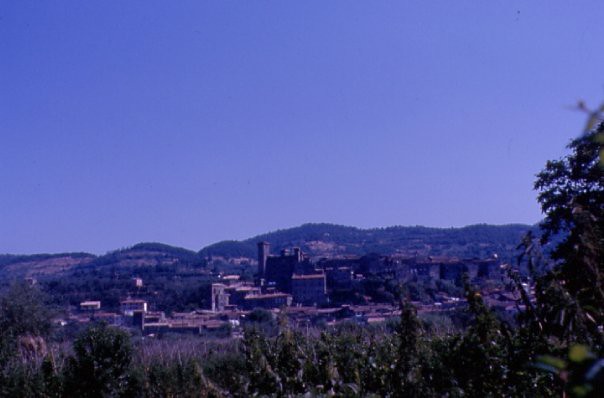The photograph captures an elevated, panoramic view of a town, likely taken from a higher or farther elevation. The sun appears to be either rising or setting, casting a bluish tint over the image, likely due to post-editing. The sky is a clear, soft blue with no clouds in sight, indicating a serene weather condition. In the foreground, green shrubberies, a hedgerow, and the leaves from a tree on the right side frame the scene, suggesting a semi-rural setting rather than a purely metropolitan one.

The town itself is semi-urban with a mix of building heights. While some structures are taller, many are of similar, moderate heights. The lack of prominent skyscrapers indicates it's not a major metropolitan area. In the background, there is a prominent hill or mountain range. The mountains appear grassy and slightly fuzzy in the silhouette, adding to the tranquility and depth of the scene.